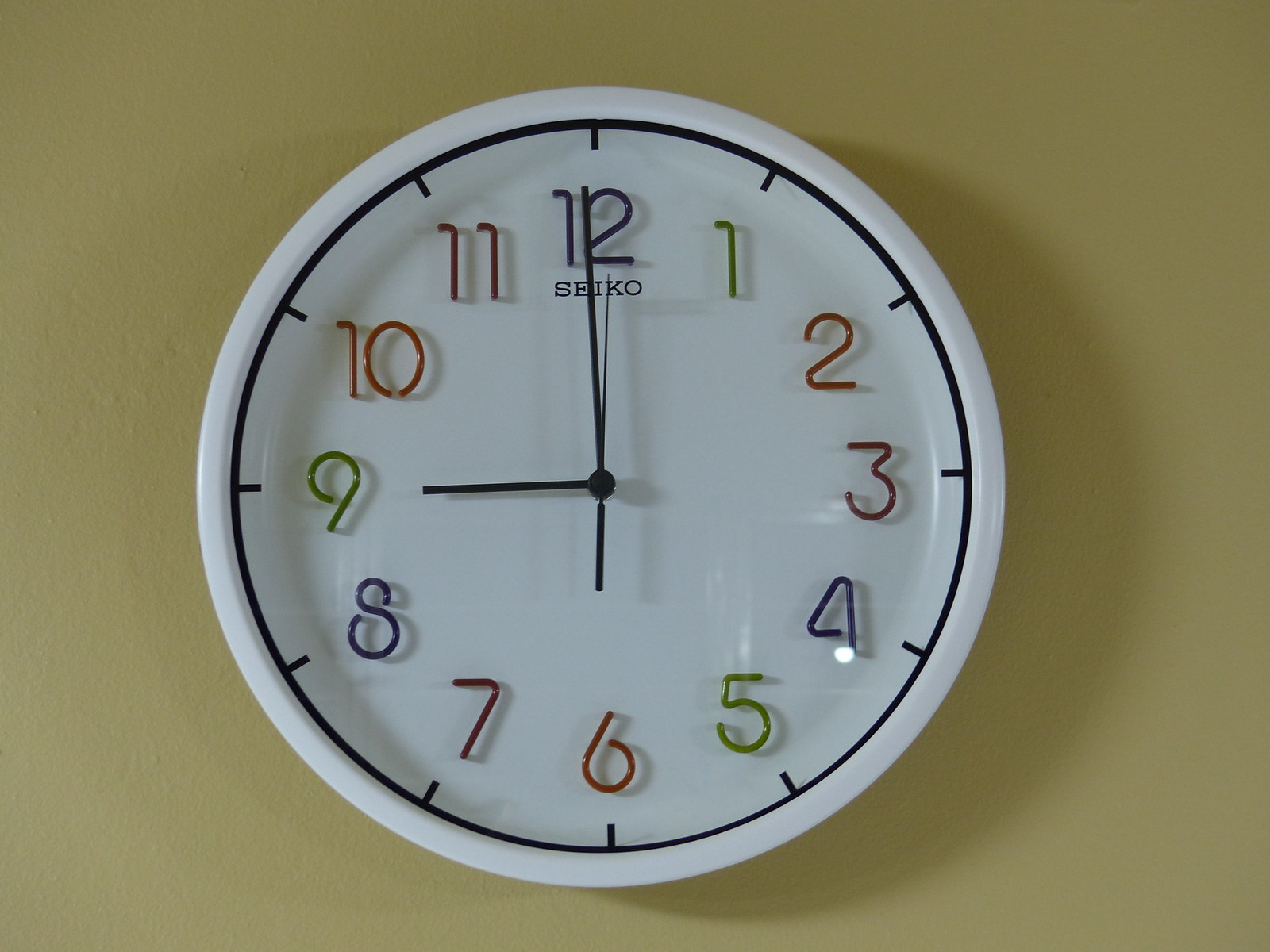The image features a Seiko clock mounted on a beige wall. The clock itself is predominantly white, including its outer rim, which is accented by a black line encircling its face. Each hour marker is characterized by a unique neon light design in various colors—1 is green, 2 is red, 3 is purple, 4 is blue, and 10 is orange. Despite their vibrant hues, the numbers are not currently illuminated. The time displayed on the clock is exactly nine o'clock.